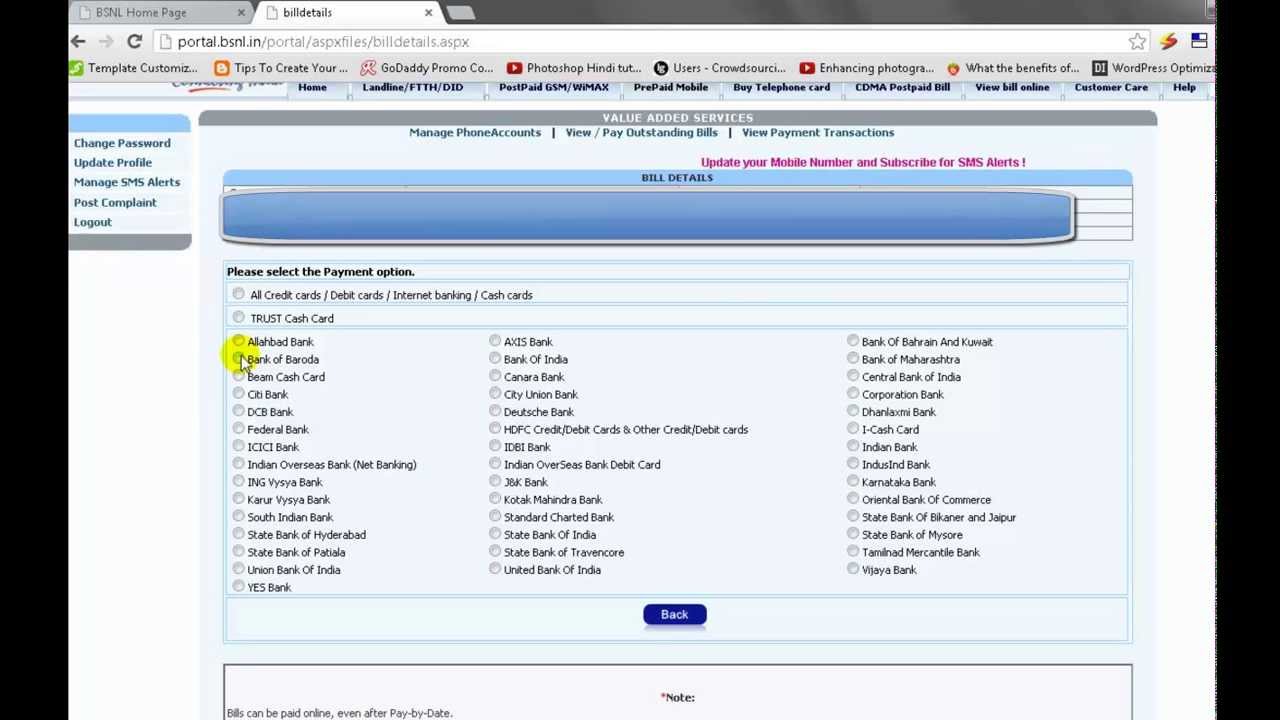A screenshot showing a web browser with two tabs open, bordered in black on either side. The tab on the right is labeled "Homepage N" and the tab on the left is titled "Bill Details," which is the active tab. The URL displayed in the address bar is "portal.bsnl.in/.portal/.aspxfiles/.billedetails.aspx." Below the address bar, the bookmark bar is visible, containing various bookmarks including "Templates," "Customized Tips to Create Your GoDaddy Promo," "Photoshop Hands," "Users," "Enhancing Photographs," and "What are the Benefits of Word Process Optimization."

The webpage being displayed is mostly white and is difficult to read due to the small font size. At the top of the page, within a gray bar, white text reads "Value Added Services." Below this, in black text, are options listed as "Manage Phone Accounts," "View Pay Outstanding Bills," and "View Payment Transactions." Further down, another option reads "Update Your Mobile Phone Number." The layout and purpose of the bookmarks raise a question about their organization, suggesting that they could be better managed within separate folders for ease of use.